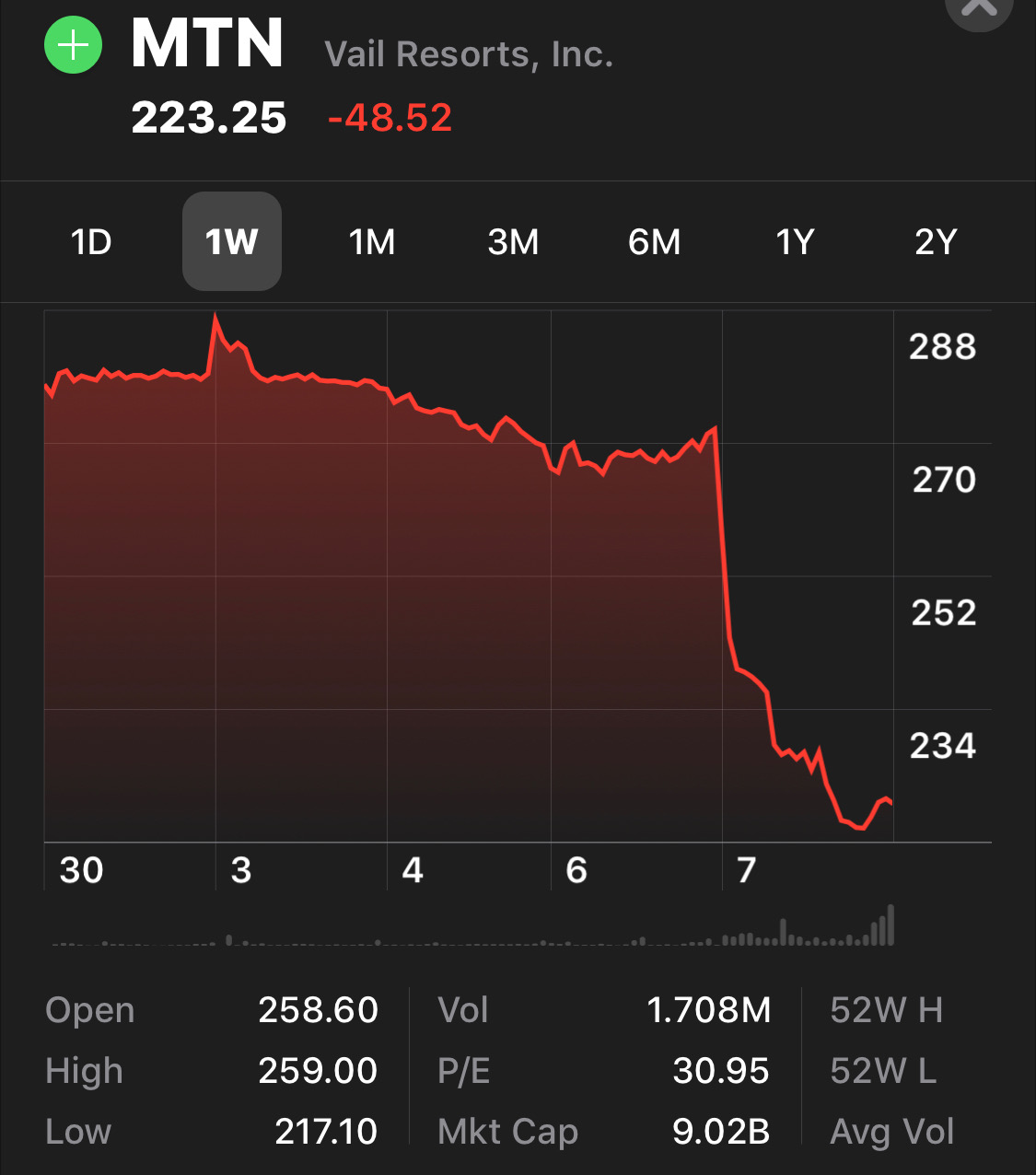The image depicts a comprehensive sales report for MTN Vale Resorts Incorporated, prominently titled at the top. The report highlights the current share value of $223.25, reflecting a decrease of $48.52. It includes a timeline with key dates: one day ago, one week, one month, three months, six months, one year, and two years. Under the two-year timeframe, the reported figures are 288, 270, 252, and 234.

Additional financial details are presented in smaller text, including:
- Opening price: $258.60
- Volume: 1.708 million shares
- Highest price: $259.00
- Lowest price: $217.10
- Market capitalization: $9.02 billion
- Price-to-earnings ratio: 30.95

These detailed metrics provide a comprehensive overview of the financial performance and market activity for MTN Vale Resorts Incorporated over various time periods.